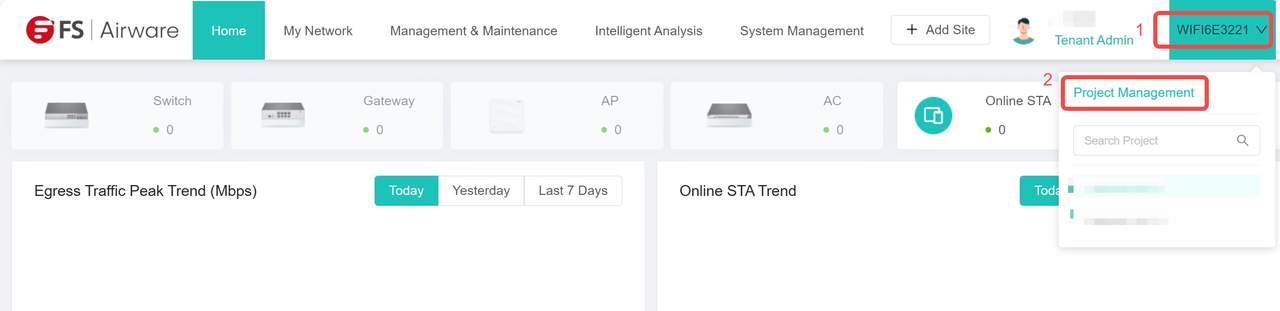The image depicts a user interface screen with various elements. 

- **Top Left Corner**: There is a white background. A small red circular icon with white lines inside it can be seen. To its right, in black capital letters, it says "FS".
- **Horizontal Bar**: Following "FS" is a horizontal bar that reads "Airwave". Adjacent to it is a bluish-green box with the word "Home" written in white letters inside.
- **Navigation Menu**: To the right, the navigation menu includes several categories. Listed sequentially, it has "My Network", "Management Maintenance", "Intelligent Analysis", and "System Management".
- **Add Site Button**: There is a small rectangular button with a plus sign and the words "Add Site", indicating a clickable element. 
- **User Profile Icon**: To the right of the "Add Site" button is a small icon depicting an image of a person.
- **Notification and Status Indicators**: On the far right, there is a bluish-green box with black numbers and letters inside. Overlapping this bluish-green box is a red rectangular box with the number "1".
- **Gray Banner**: Below these elements, a gray banner spans the width of the interface, containing various sections of information.
- **White Space**: The bottom of the page remains largely empty with significant white space, while the main information is concentrated at the top.

This detailed description outlines the layout and elements present in the interface image.